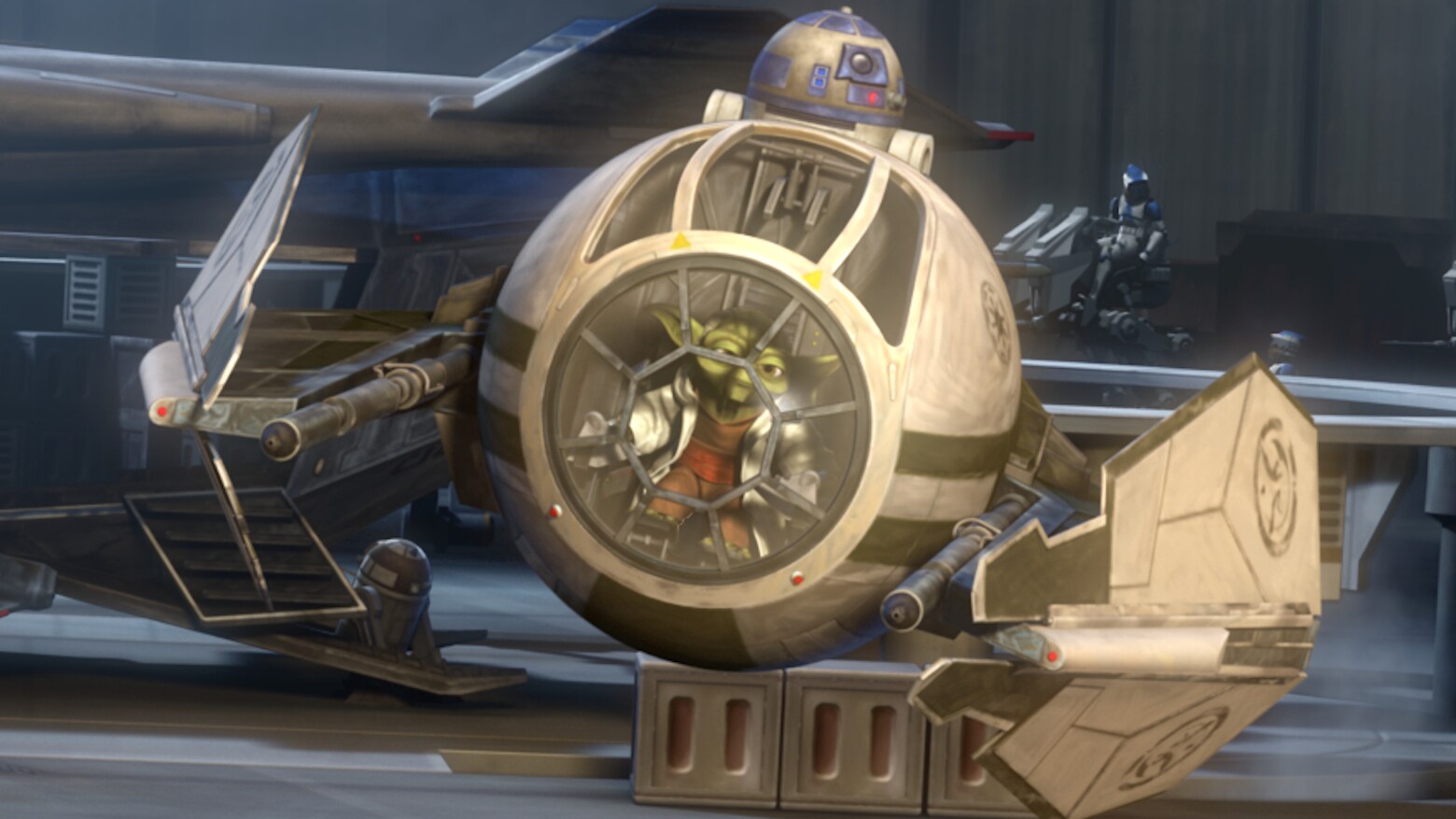This detailed animated drawing depicts a scene from Star Wars, centered around Yoda's fighter. The spaceship, primarily colored in shades of gold and dark gold, has a distinctive spherical midsection resembling a ball turret, characterized by a prominent front window. Through this window, Yoda is visible, his green head peeking out as he pilots the ship. He is adorned in a white jacket, brown attire, and a red vest, staring with an expression of intent focus. At the top of the spaceship rides a golden R2 unit, its head protruding above, serving as a co-pilot. The spacecraft's wings, which are in the process of unfolding, are notable for their circular emblems with intricate lettering and gun barrel-like extensions. The fighter rests on a platform supported by three blocks, each featuring two rectangular openings. In the background, a figure in a spacesuit can be seen, seemingly occupied with a task at a table, while other robots, rendered in gray, linger in the distance.